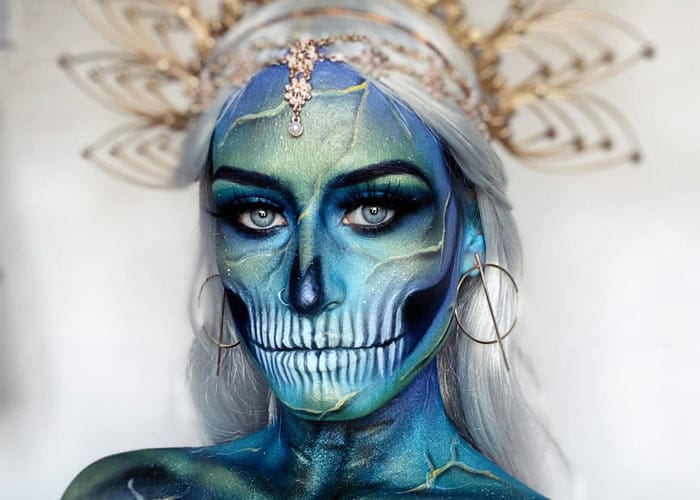The photograph features a woman meticulously adorned in an elaborate skeletal illusion created entirely with makeup. Her skin is obscured by a glossy, speckled blue paint that transitions in shades; it is darkest around her collarbones and the edges of her face, while being lighter around her neck and facial front. The makeup is accented with a black spot on her nose, around her eyes, and on her cheekbones to simulate hollows, enhancing the skeletal theme. Her mouth is artfully rendered with an x-ray-like depiction of white teeth extending across her lips. 

Blue irises framed by long, black eyelashes peer intensely at the camera, complimenting the reflective blue and green hues of her skin paint. Her silvery gray and white hair cascades down to her shoulders, partially pulled back to reveal a headpiece—a blurred but discernible crown adorned with leaf-shaped brass designs and dangling brass flowers, each crowned with a single pearl. She wears brass hoop earrings each threaded with a vertical brass dowel, and a silver nose ring graces her right nostril. The entire scene is set against a completely white, unfocused background, making her intricate and surreal appearance stand out starkly.